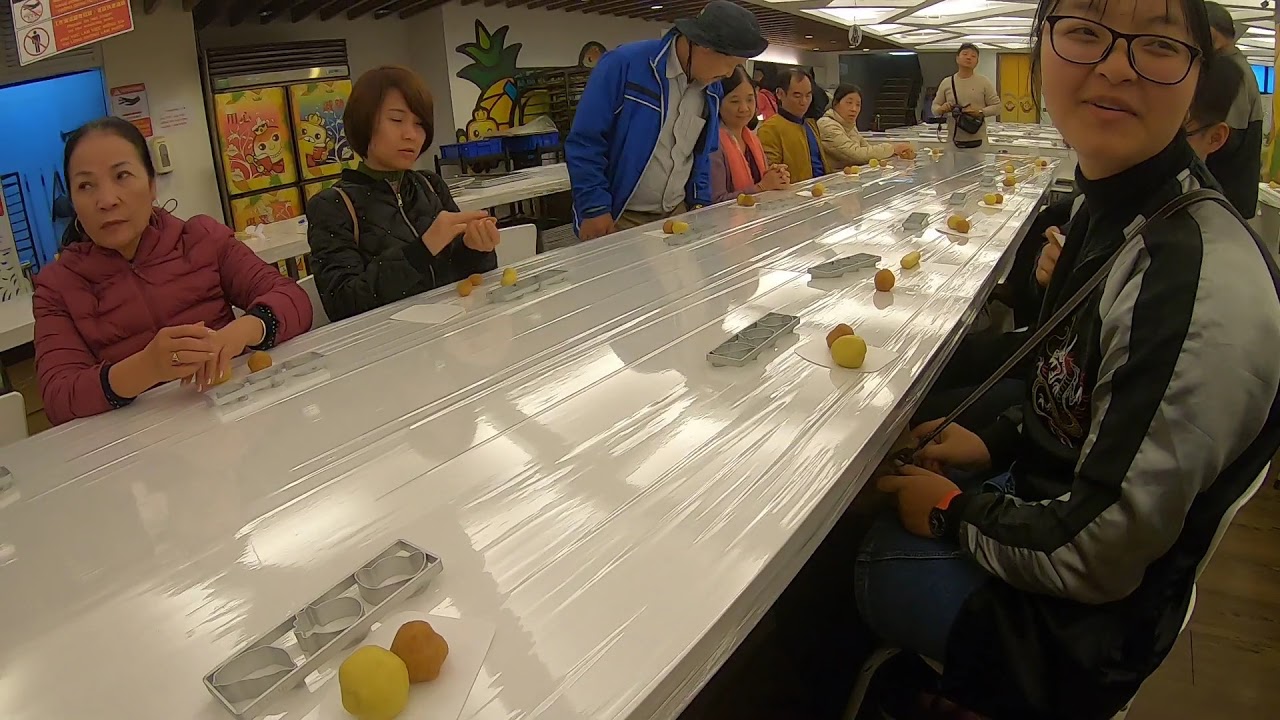The image depicts a group of Asian men and women, some seated and some standing, in an indoor setting that resembles a restaurant or cafeteria. They are gathered around a shiny white counter or long table, seated on stools, with various appetizers or collectibles in front of them. Each person has a container with three circular slots, possibly holding objects that resemble Play-Doh or dough, which some might be molding into shapes. In addition, there are brown and yellow ball-like items on the counter that appear to be part of the activity. The background features decorations including posters with pineapples and caution signs, adding to the room's eclectic decor. The people in the image, numbering around seven to ten, are dressed in various colored jackets and some wear glasses. They appear to be in a casual, engaged atmosphere, possibly preparing to eat or craft something with the items before them. The photo captures a mix of colors including light yellow, orange, black, gray, silver, fuchsia, coral, royal blue, light blue, light brown, dark green, and yellow, indicating a vibrant and lively setting.